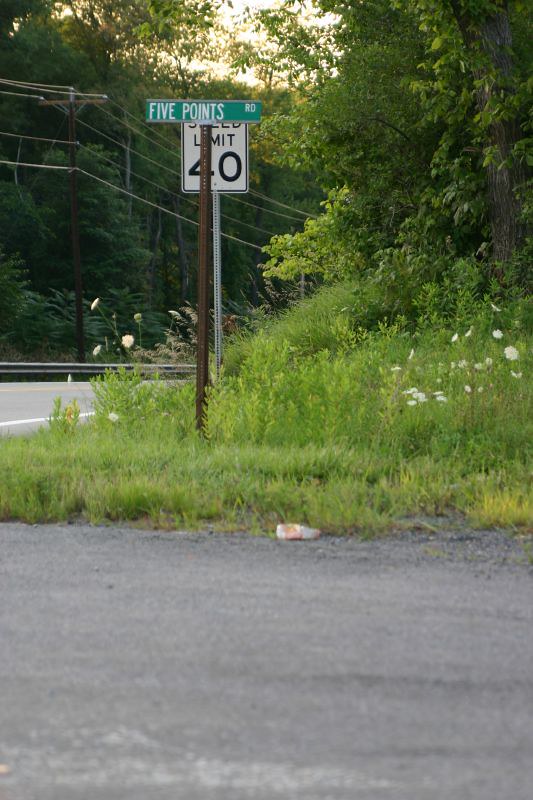In this high-quality, portrait-oriented photograph, we observe a semi-rural street corner featuring a green street sign that reads "Five Points Road" in white text. Adjacent to the street sign is a white speed limit sign indicating 40 miles per hour, with black text. Both signs are mounted on poles surrounded by tall, unkempt green grass. The road itself, paved with light grey tarmac, curves gently around the corner, marked by white edge lines. To the left of the scene, a tall power pole supports numerous horizontal power lines. Behind this pole and across the road, more trees with abundant branches and leaves are visible, adding to the density of the surrounding forest. Additionally, a light grey safety rail runs parallel to the road, contributing to the semi-rural atmosphere. Litter, including what appears to be a crushed soda bottle, is scattered at the base of the signs, along the concrete pavement. The sky is clear, with the sun high but not overly bright, casting a subtle light over the landscape.